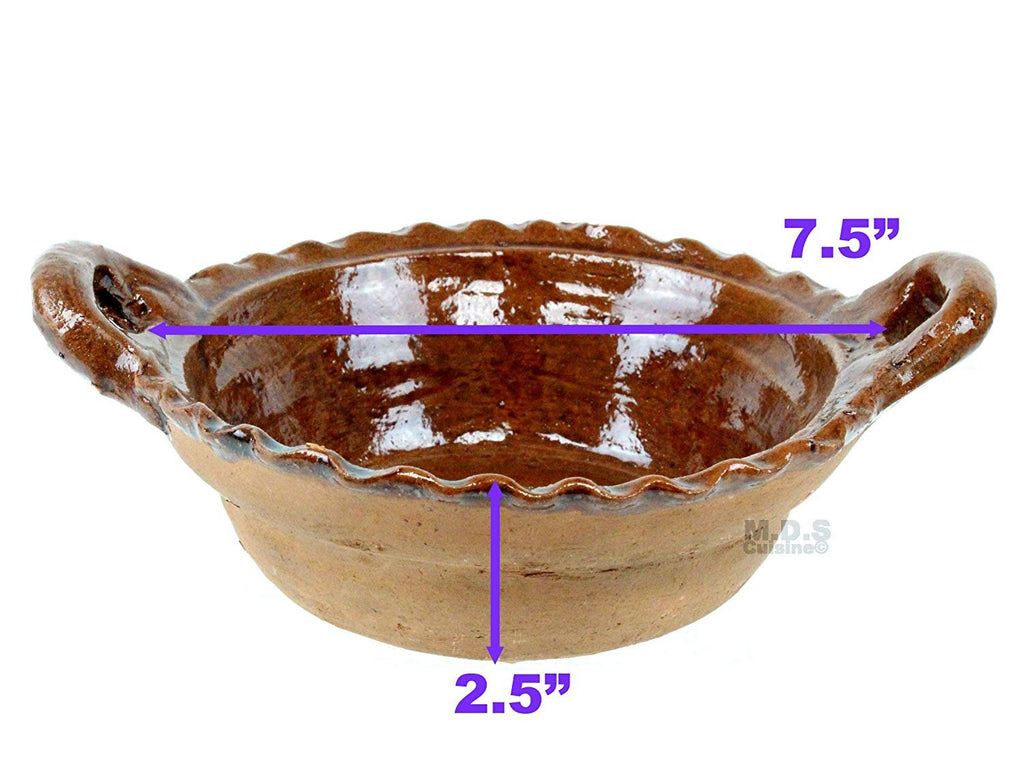The image features a handcrafted bowl made of red clay, with an overall brown hue. This circular vessel is furnished with two glossy-finished handles on either side, perfect for gripping. The interior also boasts a glossy finish and is dark brown in color. The bowl's edge is serrated with wavy patterns. Superimposed onto the white background of the photo are blue measurements: a horizontal line indicating the bowl's diameter as 7.5 inches and a vertical line noting its height as 2.5 inches. Arrows point to specific details on the bowl, enhancing the dimension annotations. Additionally, the text "NDS Cuisine" is visible on the right side of the picture, which is presented in portrait style.